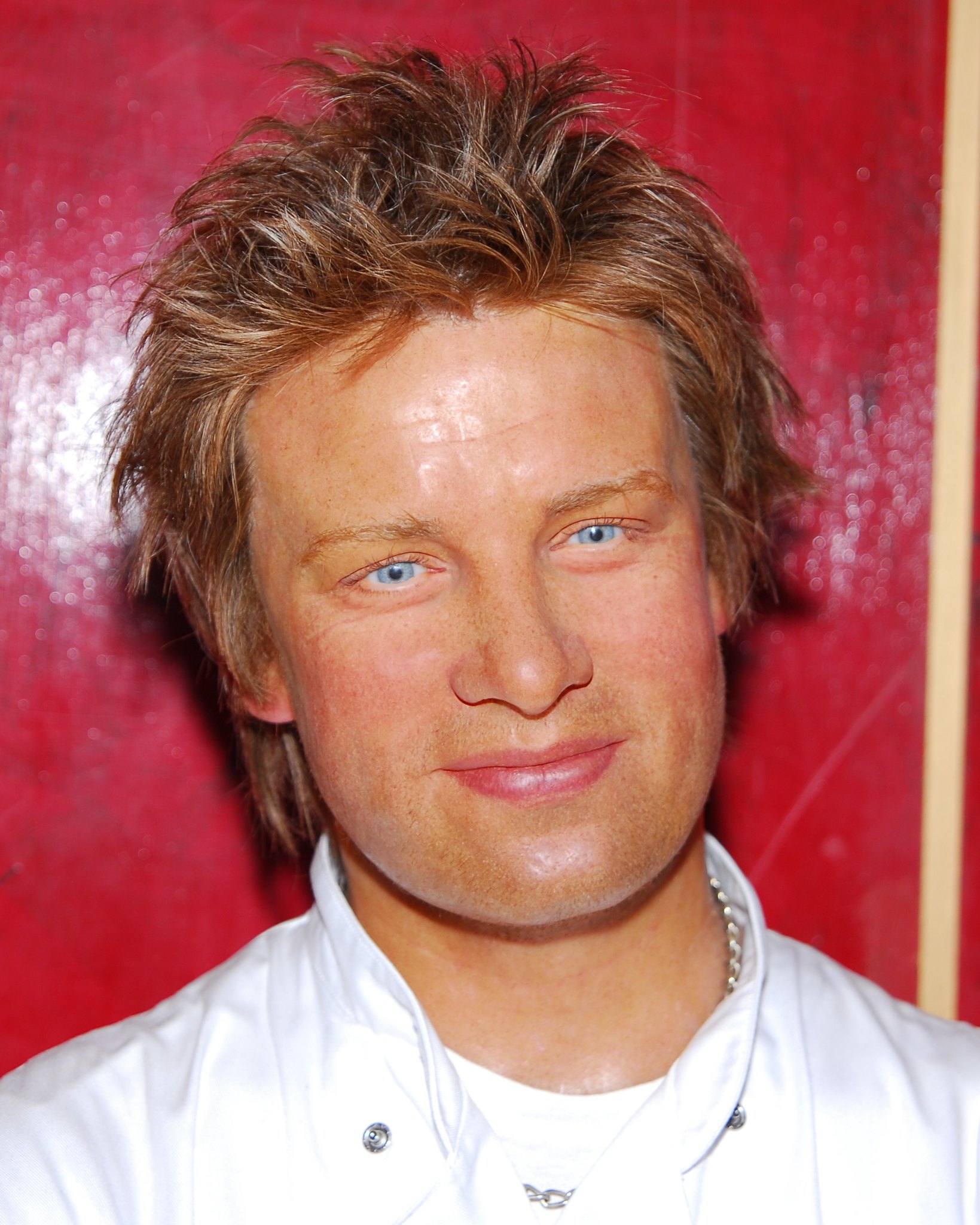This highly detailed photograph depicts a man standing in front of a glossy red wall. He bears a resemblance to celebrity chef Jamie Oliver and could potentially be a wax figure of him rather than a live person. The man is wearing a white chef’s coat with silver snaps, partially unbuttoned at the top, which reveals a white t-shirt beneath and a silver chain necklace around his neck. His red hair is styled in a slightly spiked manner on top, extending past his collar in the back, and appears a little shorter on the sides. His striking, extremely light blue eyes and numerous freckles are notable features. He has a well-defined, rectangular jawline and slightly tanned skin. The image captures him from the upper chest or neckline up, and he is smiling while looking away from the camera, giving off a professionally styled and polished appearance, with every detail of his look meticulously in place.